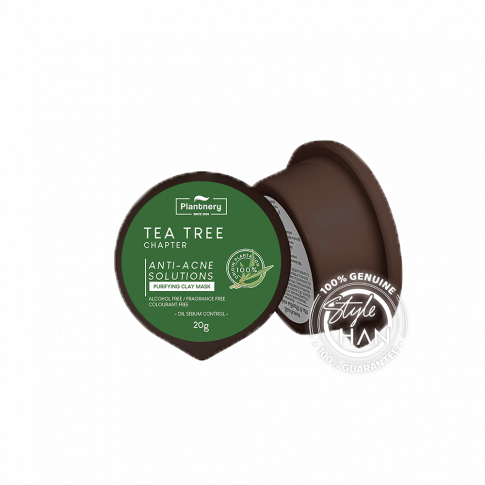The image depicts a product from the brand PLANTNERY, shown from both a front and side view. The product is contained in a small, brown tub with a green top that features a peel-off cover. The main green label prominently displays the brand name "PLANTNERY" in white against a dark green background with a swirl design. Just below the brand name, it reads "Tea Tree Chapter," followed by "Anti-Acne Solution." Additionally, there's a white rectangle on the label, within which "Purifying Clay Mask" is written. Smaller text at the bottom of the label indicates the product is "Alcohol-Free, Fragrance-Free, and Colorant-Free." The weight of the product is noted as 20 grams. The secondary side view image shows the tub leaning to its side, revealing a white label with black lettering that is not fully legible. On the lower right-hand side of the tub's green label, there's a circular logo stating "100% Genuine" at the top, "100% Guarantee" at the bottom, and "Style Han" in the center.